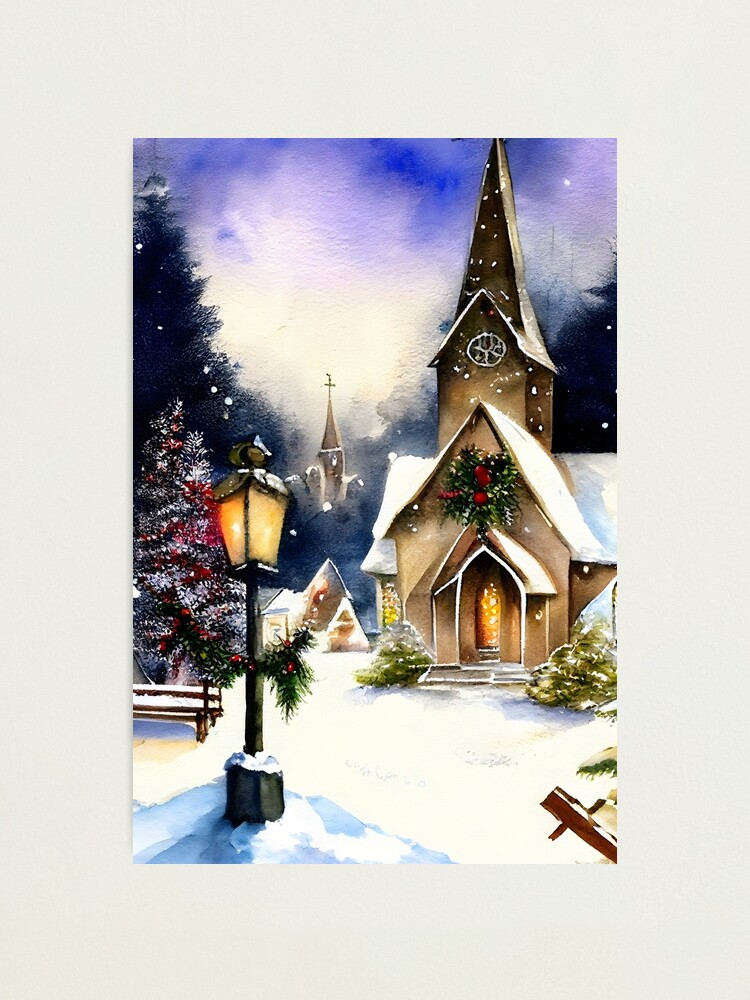This detailed image captures a Christmas card-like painting framed by a thick light gray border. Dominating the scene is a prominent brown church with a conical roof and a clock-adorned steeple. This church also features a giant wreath above its arched entryway. Snow covers the roof and ground, adding to the festive atmosphere. Red flowers and green leaves adorn shrubbery beside the church's golden door, which is accessible via a small set of stairs. In the foreground stands an old-style, illuminated black lamp post with frosted glass, also decorated with garland.

To the left of the lamp post is a tree adorned with red and white decorations. Further back in the scene, there is another church visible with a steeple capped by a cross. Trees and a wooden bench are set against a backdrop of falling snowflakes, meticulously painted as white dots scattered through the air. The sky above is a blend of blue with patches of white clouds, contributing to the serene, wintry scene.